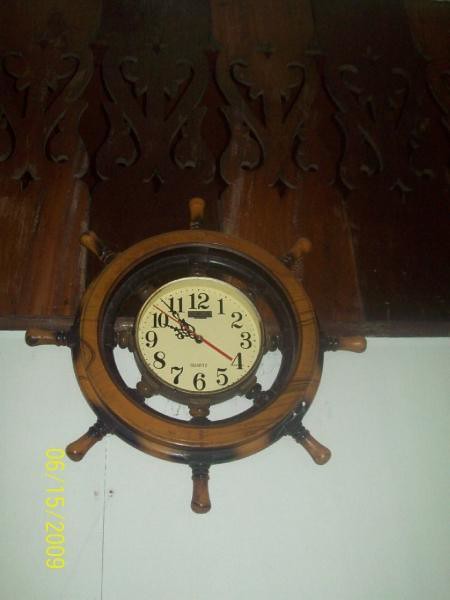Image Caption:

A beautifully crafted clock styled as a captain's wheel, featuring a medium brown finish on the outer rim and spindles that mimic the classic design of a ship's steering wheel. Each spindle has a black, fading spray-painted effect, adding a touch of rustic charm. The clock face, nestled within the wheel, boasts an off-white cream-colored base with elegant black numerals. The transparent hands are intricately designed in black, while the second-hand stands out in bright red. This nautical clock is mounted on a backdrop of individual wooden planks, each uniquely stained in rich mahogany and walnut hues, and adorned with decorative carved designs, enhancing its vintage maritime allure.